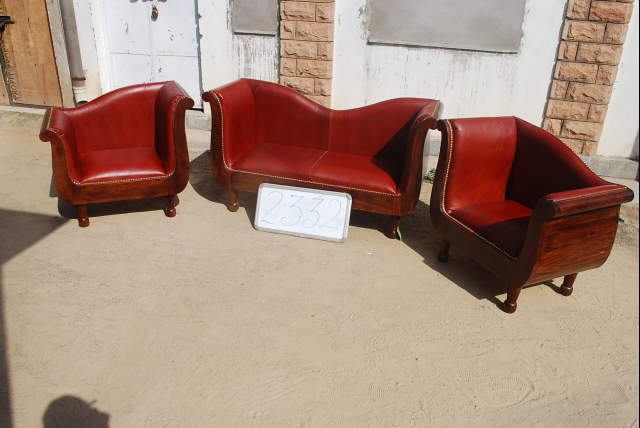The photo depicts an outdoor setting featuring a coordinated set of red leather furniture consisting of a sofa, a loveseat, and matching armchairs. These pieces are set against a backdrop of a building with white walls and interspersed brick columns, devoid of visible windows or doors. The ground appears to be pale dirt with footprints scattered across it. The furniture pieces are upholstered in smooth, brand-new red leather, characterized by their very tall backrests and armrests. The sturdy, low-to-the-ground frames are made of polished mahogany that closely matches the color of the cushions. The loveseat in the center has two cushions, with a unique backrest design that curves inward at the top, resembling a Cupid's bow. A small whiteboard placed in front of the loveseat displays the numbers "2332" in marker, and a faint shadow, possibly of a person's head, is visible in the lower left corner of the image.